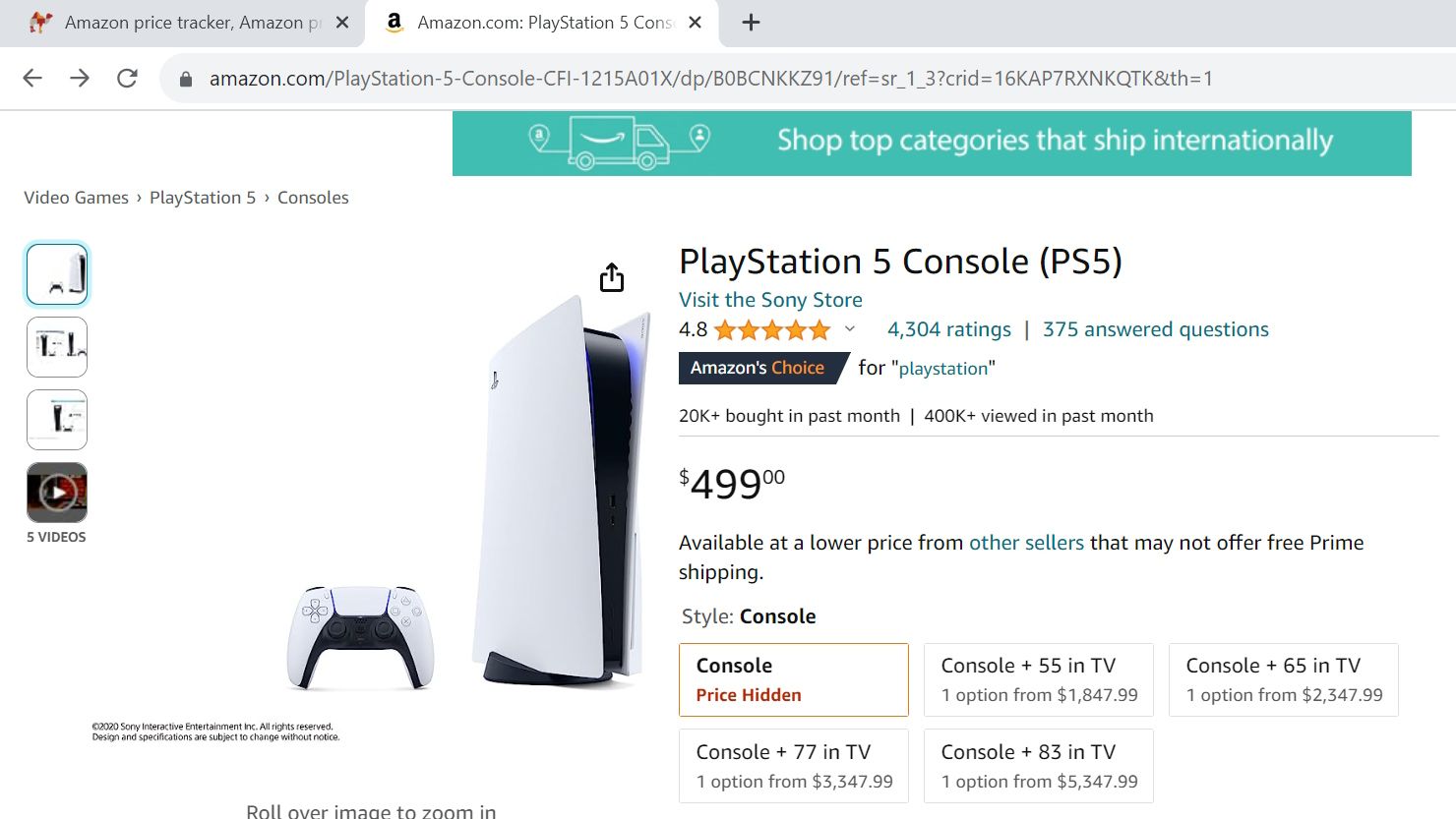The image depicts an Amazon web page, specifically showcasing the PlayStation 5 product listing. The background of the page is predominantly white, adorned with black text and occasional turquoise highlights. At the top of the page, there are two tab icons: the first reads "Amazon Price Tracker Amazon" and is not highlighted, while the second tab, which is highlighted, says "Amazon.com PlayStation 5."

The URL bar displays "Amazon.com/PlayStation5" followed by additional characters. Below the URL, an Amazon banner ad appears, promoting international shipping for top categories. Directly beneath the banner, a prominent image of the PlayStation 5 console is displayed, flanked by four smaller sub-images on the side.

The PlayStation 5 product boasts an impressive 4.8-star rating based on 4,304 customer reviews and has answered 375 customer questions. The listing is marked as "Amazon's Choice" and priced at $499. Various purchasing options are available, including different bundles such as just the console, the console with a TV, and additional configurations with TV sizes ranging from 55 inches to 83 inches.

Significant text elements include directives to "Visit the Sony store," which is highlighted in turquoise, contrasting with the predominantly black text. The PlayStation 5 console itself stands out in its sleek white and black design, serving as the focal point of the product page.